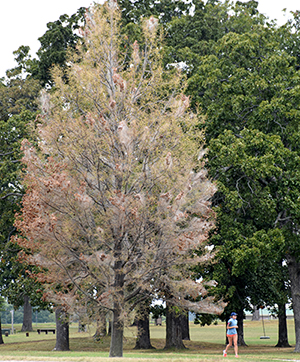The image captures a scenic view of a public park dominated by a striking large tree slightly left of center, with numerous branches extending in all directions. The tree has a unique light green and pinkish hue, with leaves that create a vivid contrast against the deep green foliage of the surrounding trees. Most of the image is filled with these trees, forming a lush canopy that reaches the top of the frame. To the right and left of this central tree, the greenery stretches upwards and nearly out of the image, with the tops of the trees almost touching the edge of the frame. In the lower right corner, a woman, dressed in a blue shirt and orange shorts with matching sneakers, is captured mid-jog, moving left to right along a path. Behind her, additional grassy areas and distant trees can be seen. Adding to the park's serene atmosphere are benches and a swing scattered around the area. The colors in the photograph—predominantly green, with splashes of white, pink, brown, and orange—create a vibrant and inviting scene.